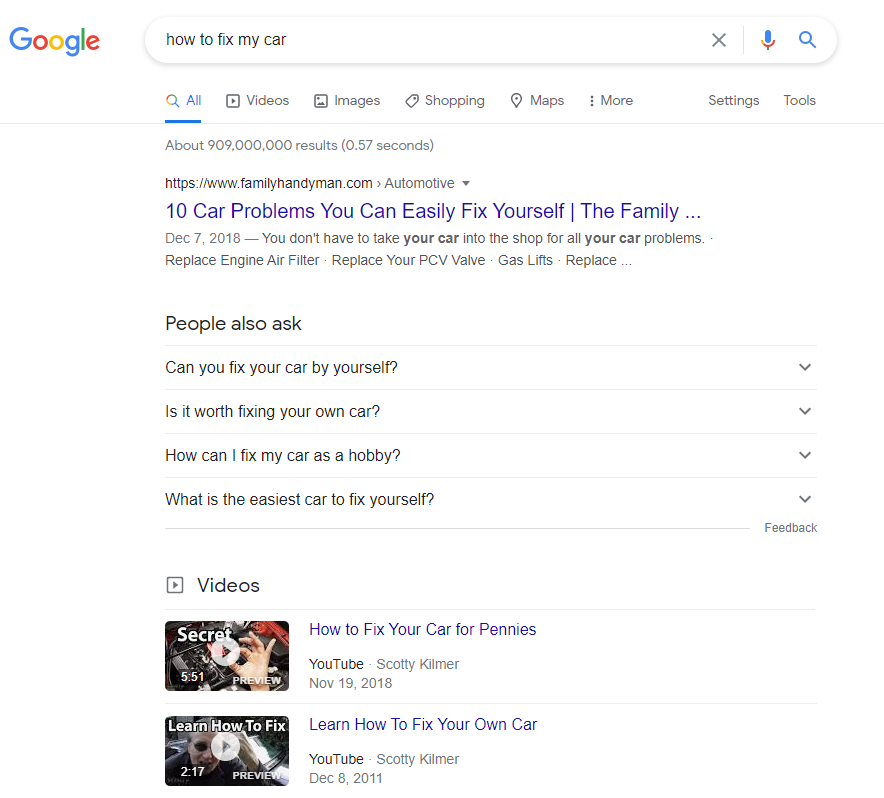The image depicts a Google search query with the phrase "how to fix my car," which yields approximately 909 million results in just 0.57 seconds. The top search result is a link to an article from familyhandyman.com titled "10 Car Problems You Can Easily Fix Yourself," emphasizing that you don't need to visit a repair shop for these common issues. Below this result, there is a "People also ask" section featuring related questions such as "Can you fix your car yourself?", "Is it worth fixing your own car?", "How can I fix my car as a hobby?", and "What is the easiest car to fix yourself?" These questions suggest slight variations of the original search that could provide additional helpful information. Further down, a series of video results appear, highlighted by two tutorials from YouTuber Scotty Kilmer. The first video, "How to Fix Your Car for Pennies", was posted on November 19, 2018, and the second, "Learn How to Fix Your Own Car", dates back to December 10, 2011.